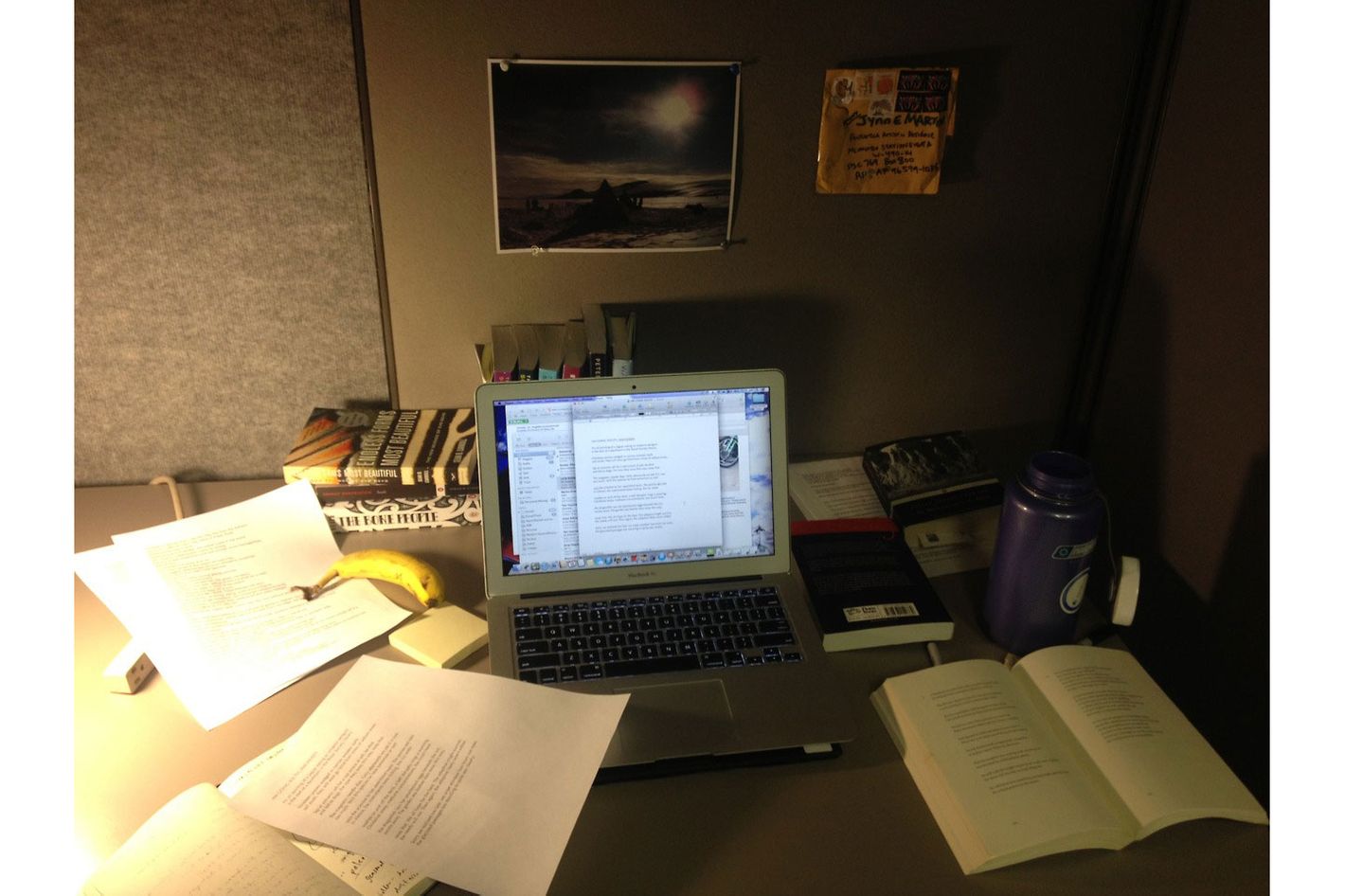The image depicts a detailed workspace setup against a light brown and speckled grey and white back wall. Attached to the wall is a white-lined picture featuring a beachfront scene with the sun and grey skies. To the left of the picture, a yellow envelope marked with black magic marker writing is visible.

At the center of the table sits a grey laptop displaying a webpage with small black font. Behind the laptop, there are two books laying flat, and another six books standing upright, although most of these are obscured by the laptop screen.

To the left, there is a yellow banana and two white sheets of paper with black writing. A cream-colored extension cord is partly visible under the papers. At the bottom left of the laptop, there are additional white sheets and some books with black font.

To the right of the laptop, an open white book with black text on both pages is placed next to a purple thermos with a black seal top. Further left, three additional books are scattered, with one being black and the others appearing to be white and grey.

The table itself is a grey desktop, providing a neutral backdrop to the varied and colorful items arranged on it.